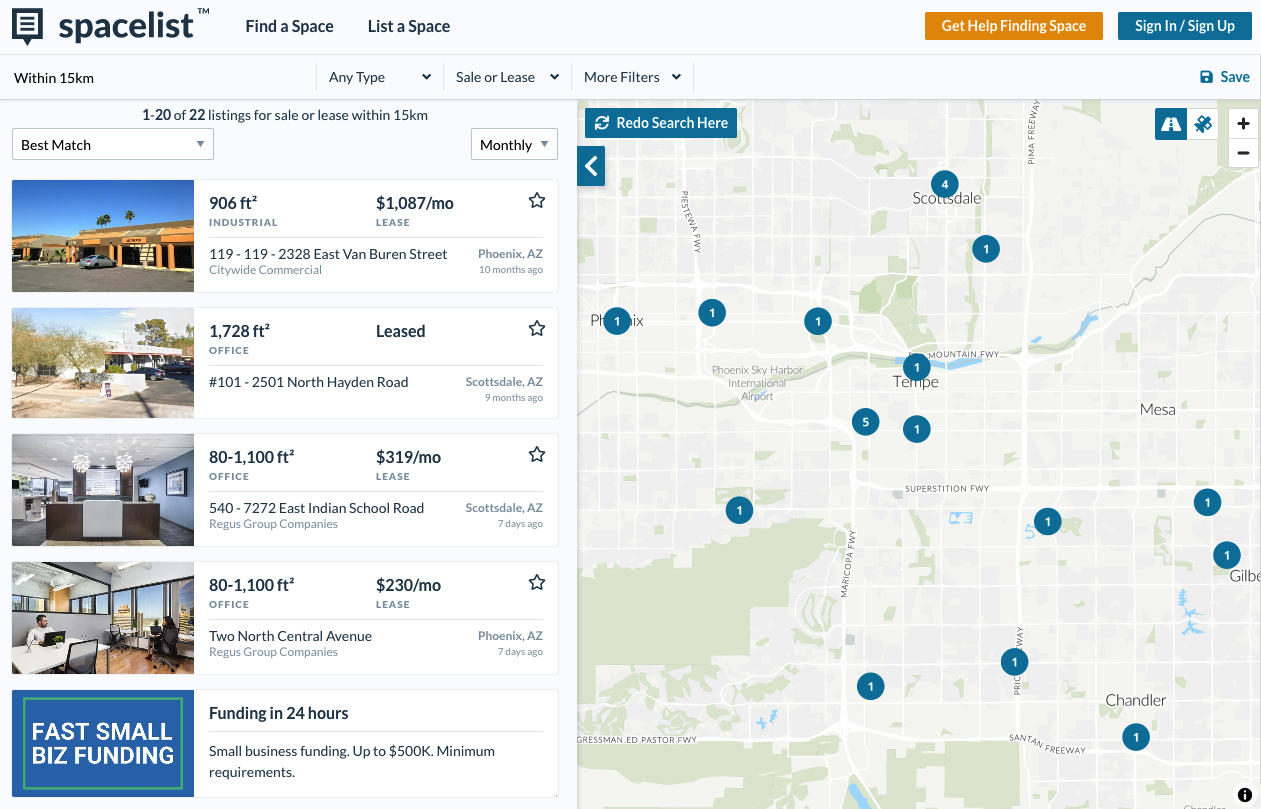The image depicts a website interface for finding commercial spaces either for sale or lease. The website's header prominently displays "SpaceList" in black font, accompanied by a small square button on the left-hand side featuring three horizontal lines.

The user has configured a search to look for spaces within a 15-kilometer radius. Various filters are available through a drop-down menu, allowing the user to specify the space type and the option to look for either sale or lease. The search results are sorted by "Best Match," revealing 22 listings within the specified area.

One notable listing offers a 906-square-foot retail building for $1,087 per month. Another listing is for a 1,728-square-foot office space available for lease. A different listing specifies a flexible space range from 80 to 1,100 square feet at a rate of $319 per month, located on East Indian School Road.

The fourth listing in focus is an industrial retail space priced at $230 per month, also with a flexible area of 80 to 1,100 square feet. This listing is provided by Regas Group Companies. The geographical locations for these spaces include two listings in Scottsdale and two in Phoenix, Arizona.

On the right side of the screen, a dynamic map displays the locations with blue dots indicating the available spaces. At the bottom of the interface, there is an advertisement for "Fast Small Biz Funding" within a blue square. The top-right corner of the interface features options for user assistance in finding a space, noticeable in an orange bar along with sign-in and sign-up options in a blue bar.

Additionally, the bottom of the interface includes a photograph of a man seated at a desk or table, possibly signifying customer support or testimonials, enhancing the website’s professional appearance.